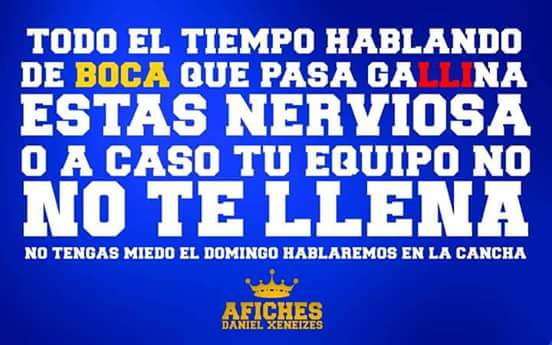The image is a Spanish advertisement featuring prominently on an ocean blue background. The text is predominantly white, with important words like "boca" highlighted in yellow and parts of "galeana" in red, creating a visually engaging contrast. The caption written in Spanish reads: "Todo el tiempo hablando de boca que pasa galeana, ¿Estás nerviosa? ¿O acaso tu equipo no te llena? No tengas miedo el domingo hablaremos en la concha,” with “no te llena” emphasized in larger text. A gold or yellow crown symbol appears at the bottom, which looks to be part of a logo that includes the name "Daniel Zizinez." The overall style and presentation suggest it is some form of advertisement or motivational messaging in Spanish.